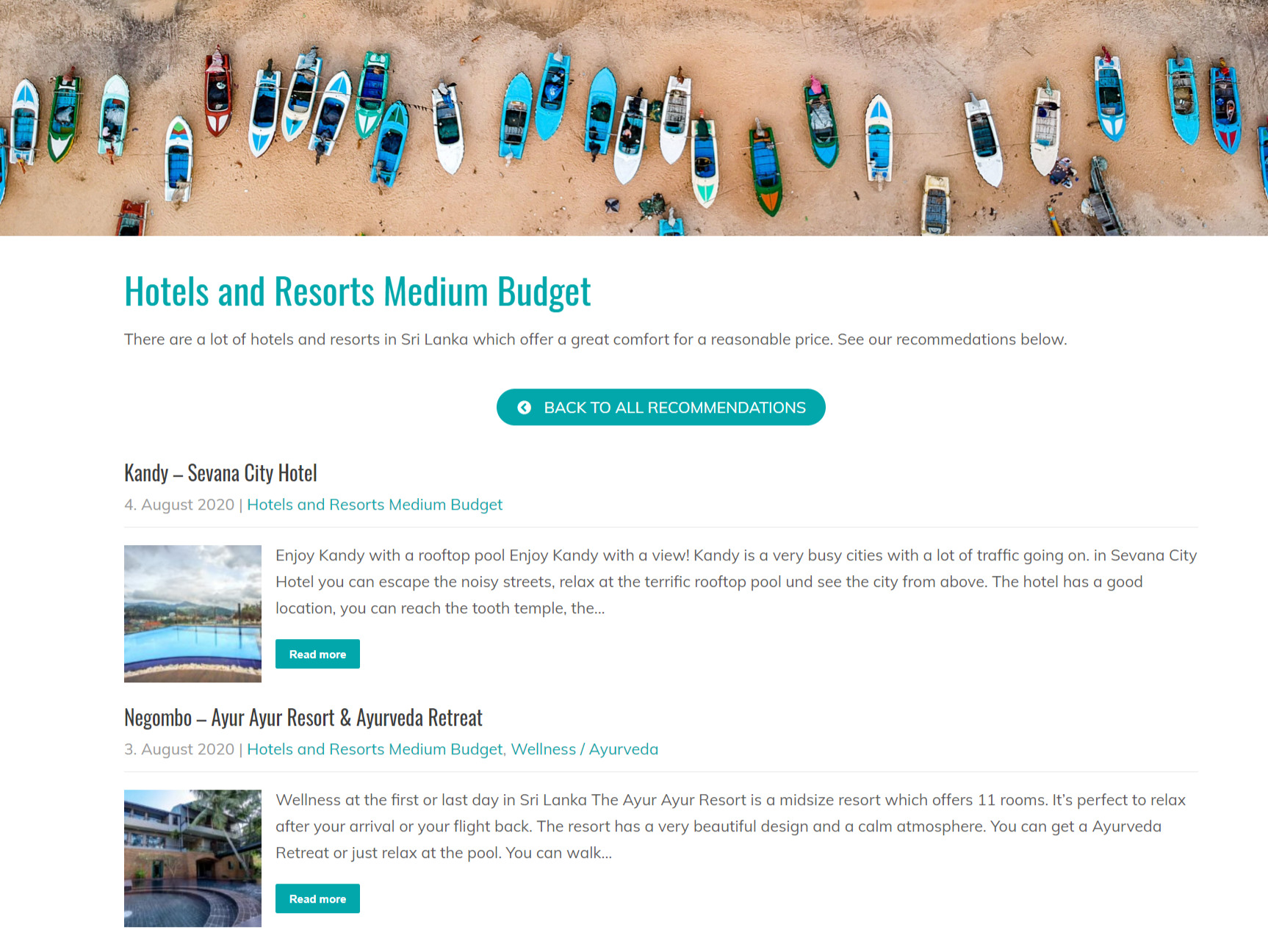**Descriptive Caption:**

This image is a screenshot of a webpage offering hotel and resort recommendations specifically tailored for travelers with a medium budget. At the top of the page, a captivating banner showcases a drone shot looking down at a collection of colorful canoes and kayaks arranged somewhat haphazardly on a sandy shore. 

Beneath the banner, in vibrant teal text, the title "Hotels and Resorts: Medium Budget" is displayed. The accompanying description reads: "There are a lot of hotels and resorts in Sri Lanka, which offer great comfort for a reasonable price. See our recommendations below." Directly below this description, a green box labeled "Back to All Recommendations" serves as a navigational aid.

The page details two distinct recommendations:

1. **Kandy Savannah City Hotel - August 2020:**
    - A medium-budget hotel and resort.
    - The accompanying image shows a slightly blurry view of the resort, featuring a pool and the distant mountains under a cloudy sky.
    - A green "Read More" button is positioned next to the picture.
    - Descriptive text provides further information about the hotel.

2. **Negombo RRR Restaurant and Aurovita Retreat - 3 August 2020:**
    - Classified under medium-budget wellness and Aurovita retreats.
    - The image presents a view of the hotel, accompanied by a "Read More" button for additional details.

The layout is designed to offer comprehensive options for budget-conscious travelers seeking comfort and quality in Sri Lanka.